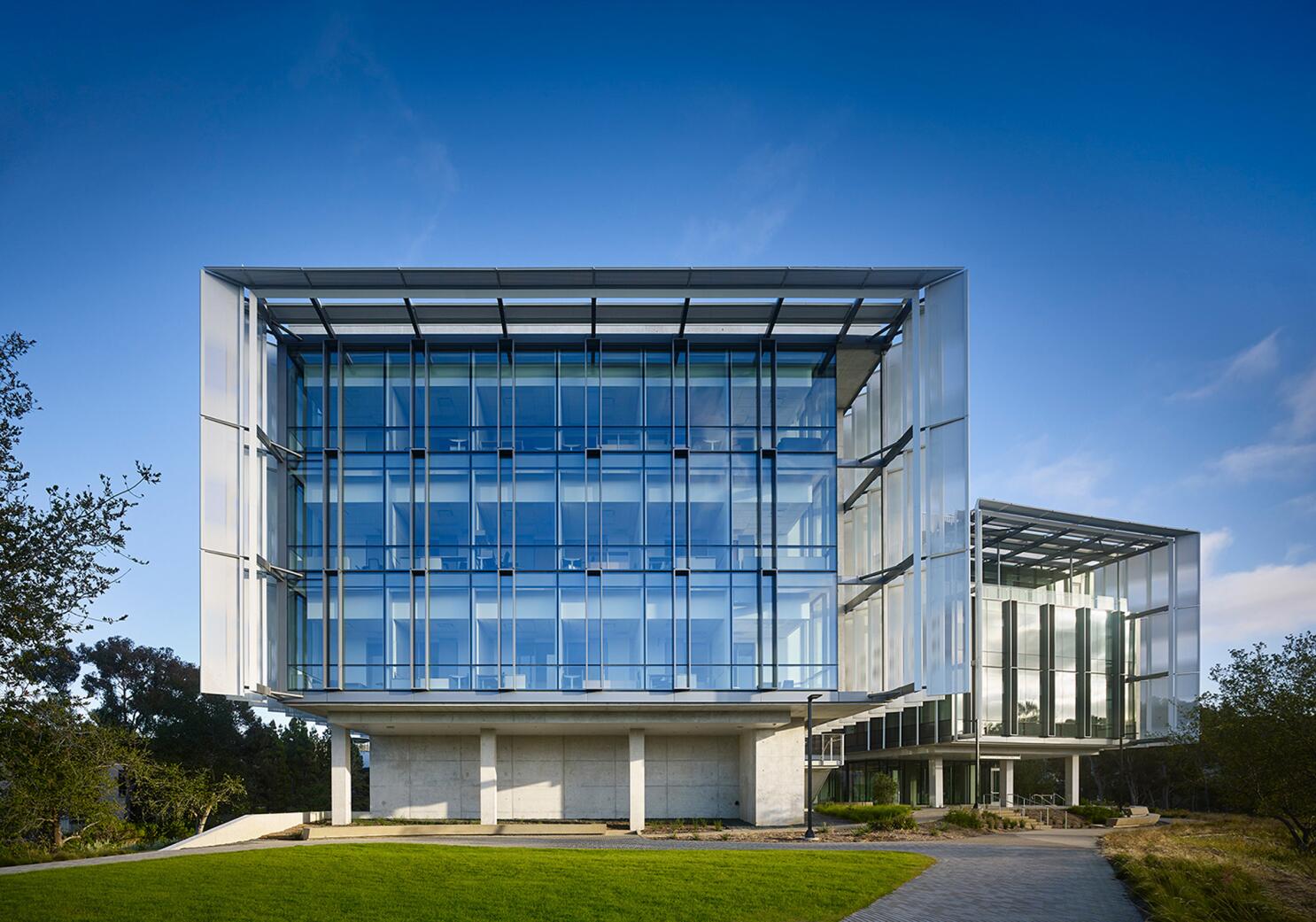This photograph features a pair of modern office buildings situated in an industrial park. Both structures are prominently made of glass, with their upper three or four stories showcasing a transparent design that allows clear visibility into the interior offices, filled with cubicles and chairs. The buildings, which possess a square, almost cube-like architectural style, rest on concrete bases, augmented by some brick pillars and detailed grid work holding the construction together.

The foreground of the image is adorned with a well-kept green lawn and scattered trees, while a sidewalk with miniature streetlights leads up to both buildings, emphasizing the modern and organized landscape around them. The background reveals a blue sky with white clouds, enhancing the open and isolated atmosphere of the scene, indicating that the office complex is likely for a wealthy company seeking a unique and spacious environment. Notably, one of the buildings features a large, box-like projection, contributing to its distinct and striking architectural flair.